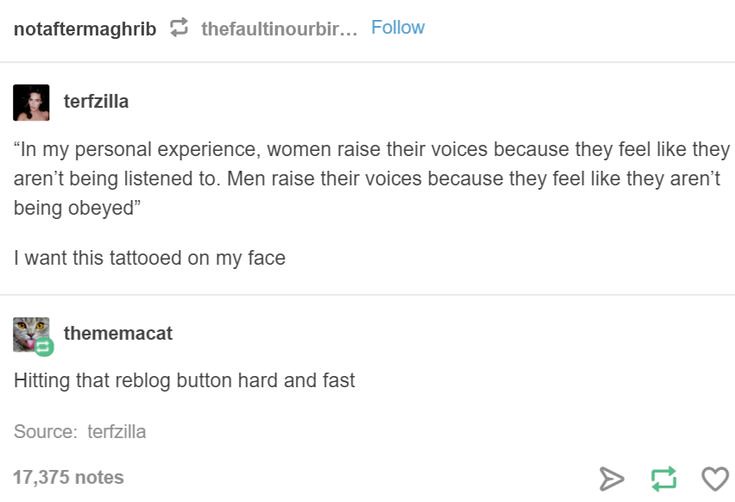The image is a screenshot from an unspecified social media app, showcasing two user profiles engaged in a discussion. The screenshot features multiple lines of small black text against a gray background. At the very top, it reads "Not after Magrib" followed by "Follow" in blue. The first post is made by a user named Turfzilla, whose profile thumbnail is a picture of a woman. Her post states, "In my personal experience, women raise their voices because they feel like they aren't being listened to. Men raise their voices because they feel like they aren't being obeyed. I want this tattooed on my face." The second post is from TheMamaCat, whose profile thumbnail is a cat. She agrees with Turfzilla, humorously adding, "My cat hitting that reblog button hard and fast." The post by Turfzilla has garnered significant engagement, with 17,375 notes. The only color in the image comes from a green repost button, while other icons, including one resembling a paper plane and another with two arrows pointing left and right, are visible at the bottom right.